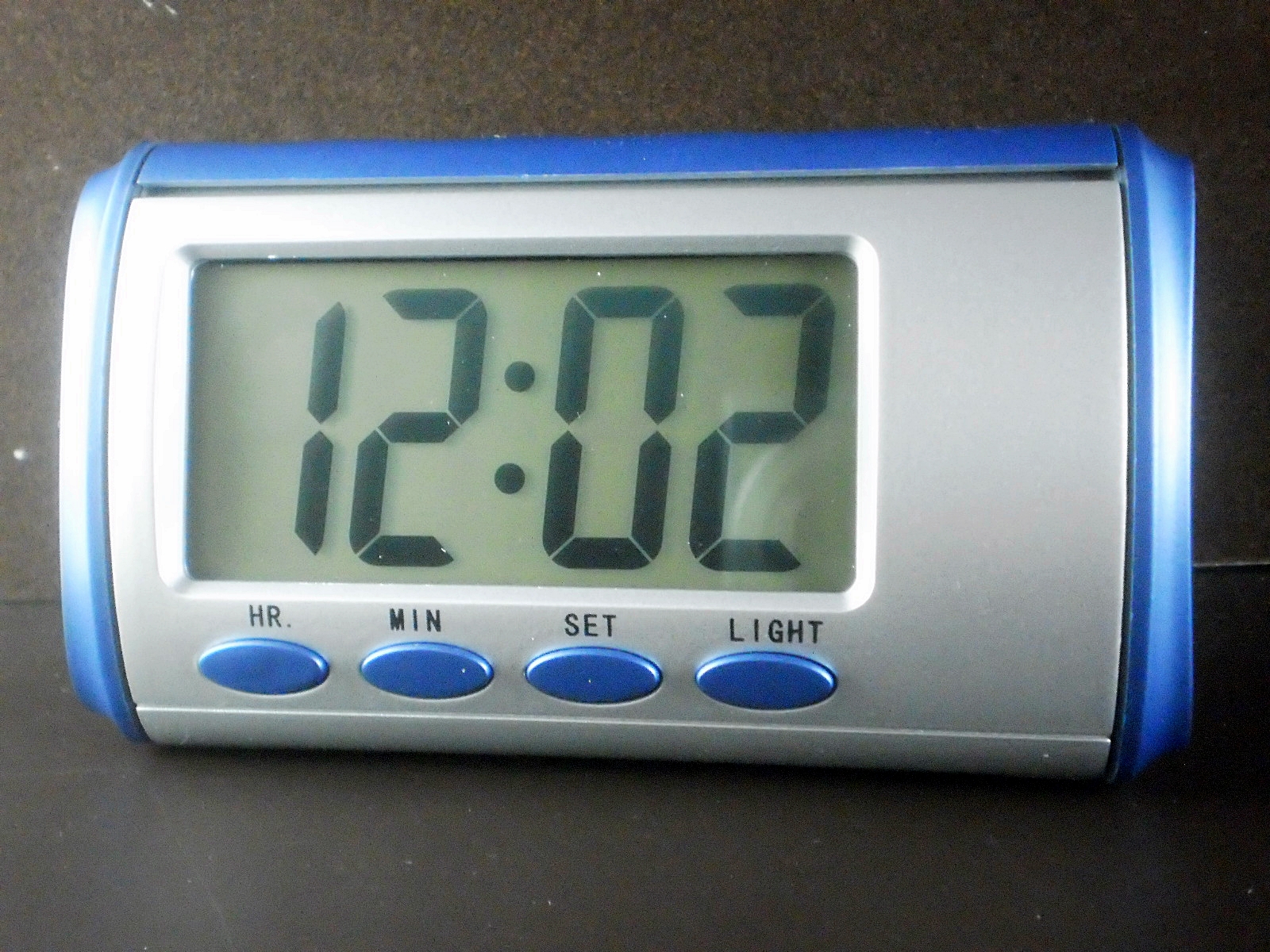The photograph, taken indoors, captures a small plastic alarm clock positioned on a dark brown table. The table's rich hue is echoed by the similarly dark brown wall in the background, creating a cohesive and warm setting. The focus of the image is the alarm clock, which features a bright blue casing along its sides and top, contrasting vividly with the table and wall. The front panel of the clock is silver, accentuated by blue buttons labeled in black writing. The four buttons are marked HR, MIN, SET, and LIGHT. The digital display, showcasing the time 12:02 in black digits, stands out against a slight greenish background provided by the LCD screen. This detailed composition highlights the alarm clock's functionality and design within its indoor setting.